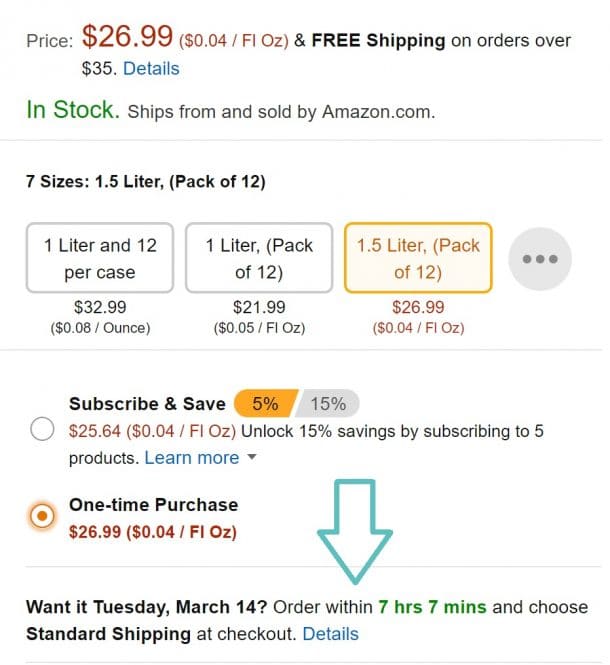The image is a detailed screenshot of product pricing from Amazon. At the top, it prominently displays the price of $26.99 for 0.04 fluid ounces, with a note indicating free shipping on orders over $35.

Just below that, in green text, the availability status reads "In Stock" and specifies that the item "Ships from and sold by Amazon.com."

Further down, the product offers a choice of seven sizes, with a particular focus on a 1.5-liter option available in a pack of 12. Three rectangular selection boxes are shown, with the first two in white. The first box indicates "1 liter, 12 per case" with a price of $32.99, and the second box shows "1 liter, pack of 12" priced at $21.99. The third box, highlighted to stand out, represents the 1.5-liter, pack of 12 option, priced at $26.99.

Below these options, there is a "Subscribe & Save" section, offering a discounted price of $25.64 if subscribing to five products for a 15% savings, accompanied by a blue link to "Learn more."

Next, the image showcases the "One-time purchase" option, highlighted with a round button, listing the price as $26.99. Adjacent to this, a large white arrow outlined in green points downwards, with a prompt stating, "Want it Tuesday, March 14? Order within 7 hours 7 minutes and choose standard shipping at checkout," followed by a link labeled "details."